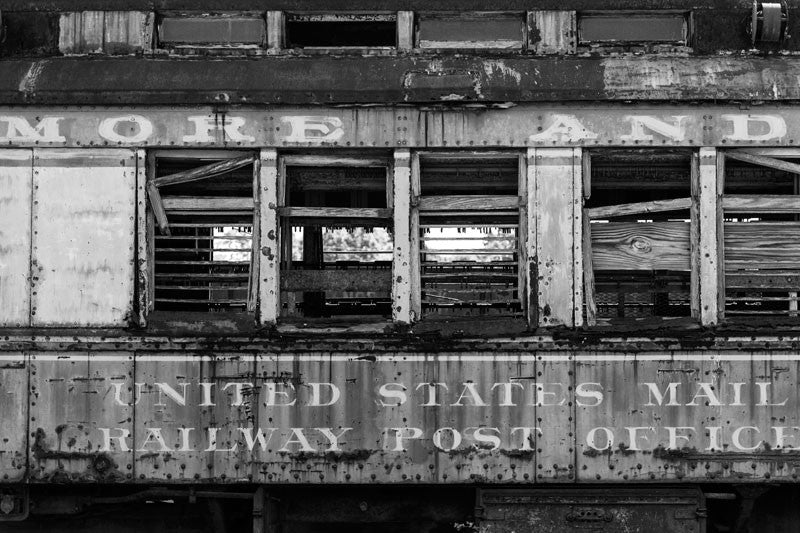This black-and-white photograph captures a severely dilapidated railway carriage, revealing a poignant image of abandonment and decay. The carriage, rusted and neglected, bears the faded inscriptions "United States Mail Railway Post Office" prominently displayed on its side. Above these words, the text "More And" appears, though incomplete due to the framing of the photograph. The bottom portion of the image is enveloped in darkness, emphasizing the extent of deterioration. The carriage's metalwork and rivets are corroded, adding to the sense of neglect. There are five full windows in view, with what's left of blinds and wooden louvers in various states of disrepair, while five more partial windows can be seen above, separated by a slanting roof line. Some windows are boarded up with wooden panels or steel plates, reflecting attempts to seal them as they began to fall apart. Notably, the fourth window from the left features a makeshift pine panel wedged into the sill. This evocative image serves as a testament to the passage of time and the forgotten era of the railway mail service.